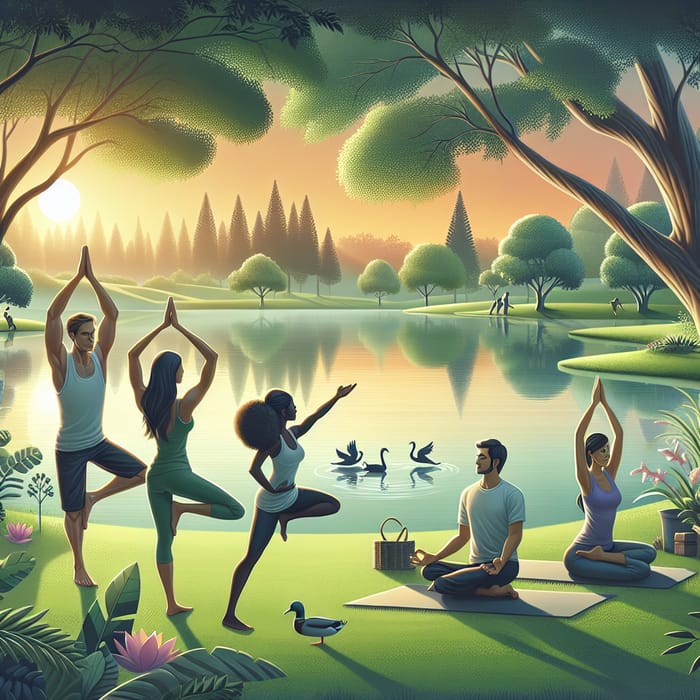This cartoon illustration depicts a serene park scene around a lake during sunset. The sky is awash with orange hues, reflecting the setting sun. Around the lake's green grass perimeter, several people are engaged in various yoga poses. In the foreground, vivid pink flowers with green leaves add color to the scene. On the right side, one woman in purple sits cross-legged on a yoga mat with her hands raised above her head. Nearby, a man with a basket beside him sits in a pose with his hands on his knees, and a duck stands close by. At the center, a woman in white stretches her arms out, while another woman balances on one leg with her hands over her head. A man in a white tank top also stretches his hands over his head. The calm lake hosts three swans, their serene reflections visible in the water. The background features rows of trees and their branches extending to frame the top of the image, creating a lush, natural canopy. Additional people are seen in the distance, further enhancing the tranquil, communal atmosphere of the park.